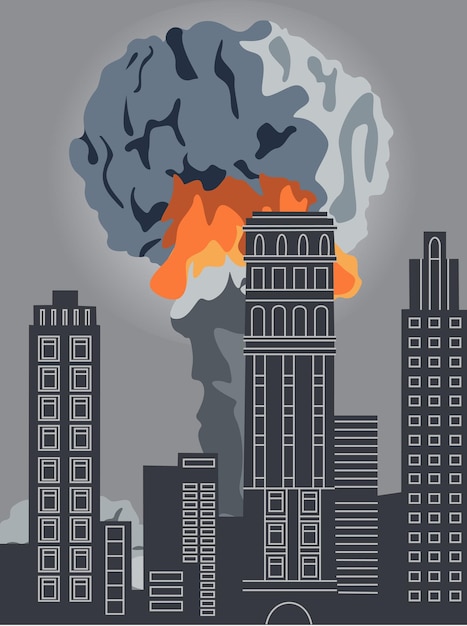This digital artwork illustrates a cityscape under a grey sky, dominated by a towering mushroom cloud suggestive of a massive explosion or nuclear event. The city is depicted with tall skyscrapers, primarily black with simplistic white outlines for windows, enhancing their silhouette against the chaotic background. The explosion's mushroom cloud rises ominously behind the buildings, starting with a dark grey pillar of smoke at the base. A vibrant orange and yellow ring of flames encircles the middle, adding stark contrast to the predominantly monochromatic scene. The top of the mushroom cloud expands into a large grey puff, completing the explosive imagery. The artwork's flat, shaded style reinforces the sense of a stark, catastrophic event unfolding within an otherwise calm urban environment, evoking scenes reminiscent of major metropolises like New York or San Francisco.